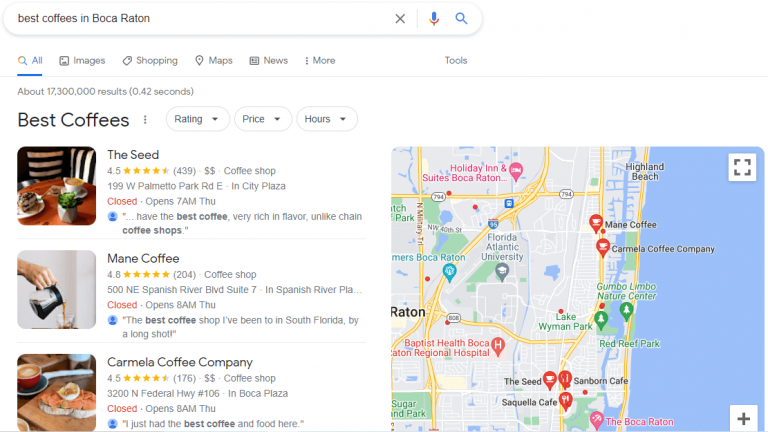The image depicts Google search results for "best coffee beans in Boca Raton" on a white background. At the top left, a search bar spans the width, containing the query "best coffee beans in Boca Raton". The search bar has a gray edge and features a microphone icon on the right, followed by a magnifying glass search icon. Beneath the search bar, navigation options such as All, Images, Shopping, Maps, News, More, and Tools appear in a row, with "All" highlighted in blue and underlined.

Below the navigational options, the search results indicate approximately 17.3 million results found in 0.42 seconds. The results include filtering options for rating, price, and hours. The top search results begin with "The Seed," which is visually represented by an image of a table laden with plates and food. Following this, "Main Coffee" appears, accompanied by an image of a hand pouring coffee. Next is "Carmelo Coffee Company," illustrated by a photo of a table with coffee cups and plates. Each listing includes star ratings and typical search result details.

To the right of the search results, a map showcases the area around Boca Raton, with the ocean depicted on the right and land with city markers on the left. Numerous pins on the map indicate the locations of various coffee shops.